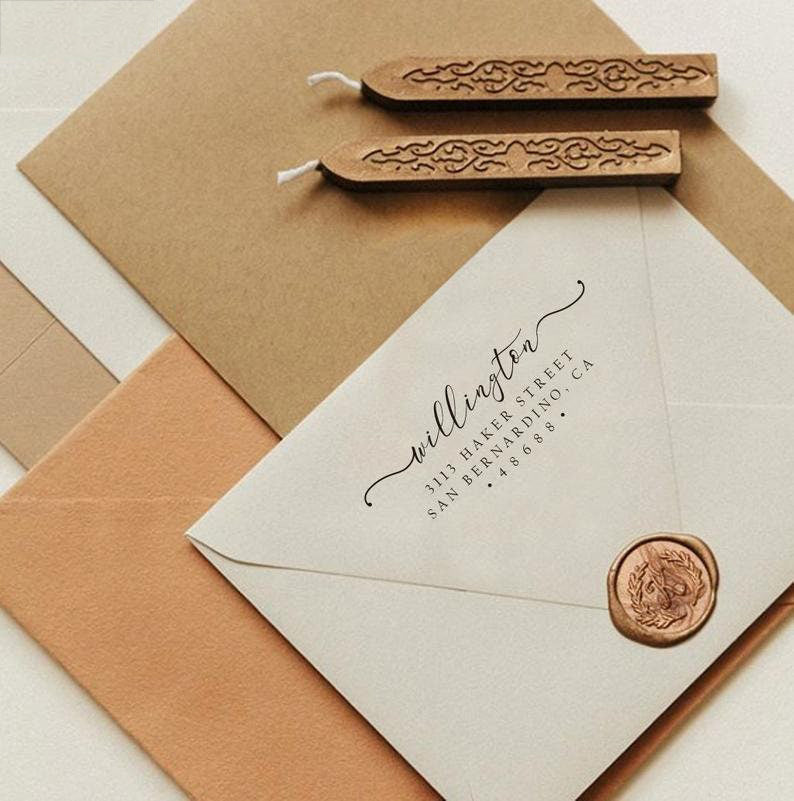This image features a detailed arrangement centered around a light gray envelope that is slightly tilted to the left. The envelope bears elegant cursive black text reading "Wellington," with the address "3113 Acre Street, San Bernardino, CA 48688" printed in uppercase black letters below it. Distinctively sealing the flap of the envelope is a gold wax stamp bearing grain depictions. Above this main envelope, there are two vertically aligned candles, each shaped like a long rectangle and tapering to a point where the wicks are located; these candles feature imprints on their bodies. In the background, several other envelopes can be seen: a brown envelope located at the top and a light orange one positioned near the bottom. The entire setup conveys a formal and sophisticated ambiance, reminiscent of materials used for special occasions such as wedding invitations.